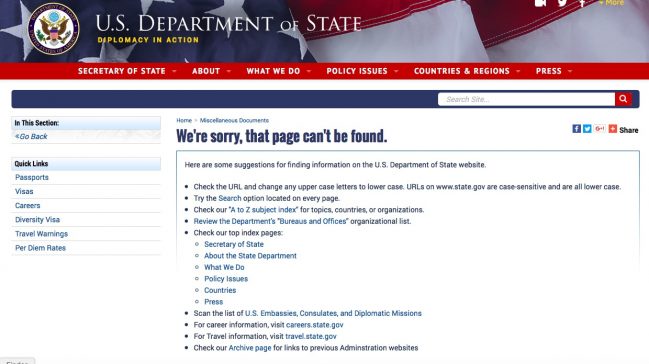The image displays a web page with a white background. At the top, there's an American flag and a round seal featuring an eagle, with a blue dot above it and an American flag in the center. The seal reads "U.S. Department of State, Diplomacy in Action," with "Diplomacy in Action" highlighted in yellow.

Beneath the seal, a red navigation bar displays links labeled "Secretary of State," "About Us," "What We Do," "Policy Issues," "Countries and Regions," and "Press." A long blue line separates this section from the search bar, which has a red end with a magnifying glass icon.

On the left side, a small blue box is followed by a white box with a "Go Back" button. Another blue box labeled “Quick Links” is present, along with white boxes offering access to "Passports," "Visas," "Diversity Visa," and "Per Diem Rates," each accompanied by a camera icon and possibly warnings.

At the bottom, there's a small-print message stating, "We're sorry, that page can't be found." To the right, icons for Facebook, Twitter, and other social media platforms appear, along with a "Share" option.

A blue-outlined section provides suggestions for finding information on the U.S. Department of State website, listing five bullet points followed by a dropdown menu with four more suggestions.